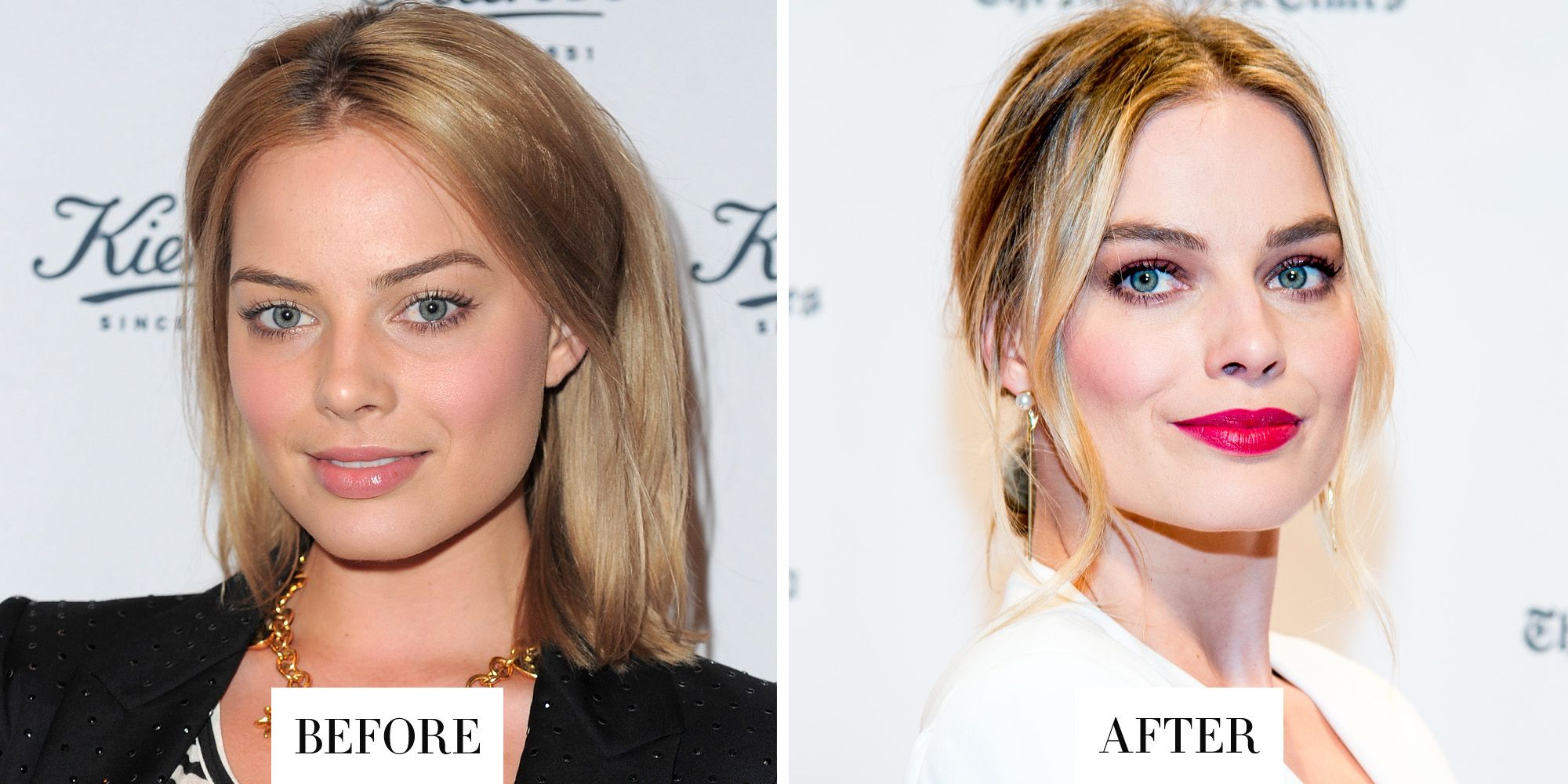The image features two side-by-side photographs showcasing what appears to be a before and after comparison of the same actress, possibly Margot Robbie. In the left photograph, the actress is depicted as younger, perhaps in her early twenties, with dirty blonde hair, blue or gray eyes, pink lipstick, and makeup. She's dressed in a black top and adorned with a gold necklace, standing against a backdrop that includes a sign reading something like "K.I.E" and a date, possibly 1901 or 1981.

The right photograph presents her at a later stage in life, seemingly in her mid-thirties. Her hair remains dirty blonde but is straighter and appears more spindly. Her eyes are now a hint more green, and she wears very vibrant, painted-on red lipstick. Her face is notably pale with slight blushing. She is dressed in a white top, accessorized with pearl earrings, and her demeanor appears more mature. Both photographs highlight the actress's evolving appearance over time while providing subtle details and background elements for context.